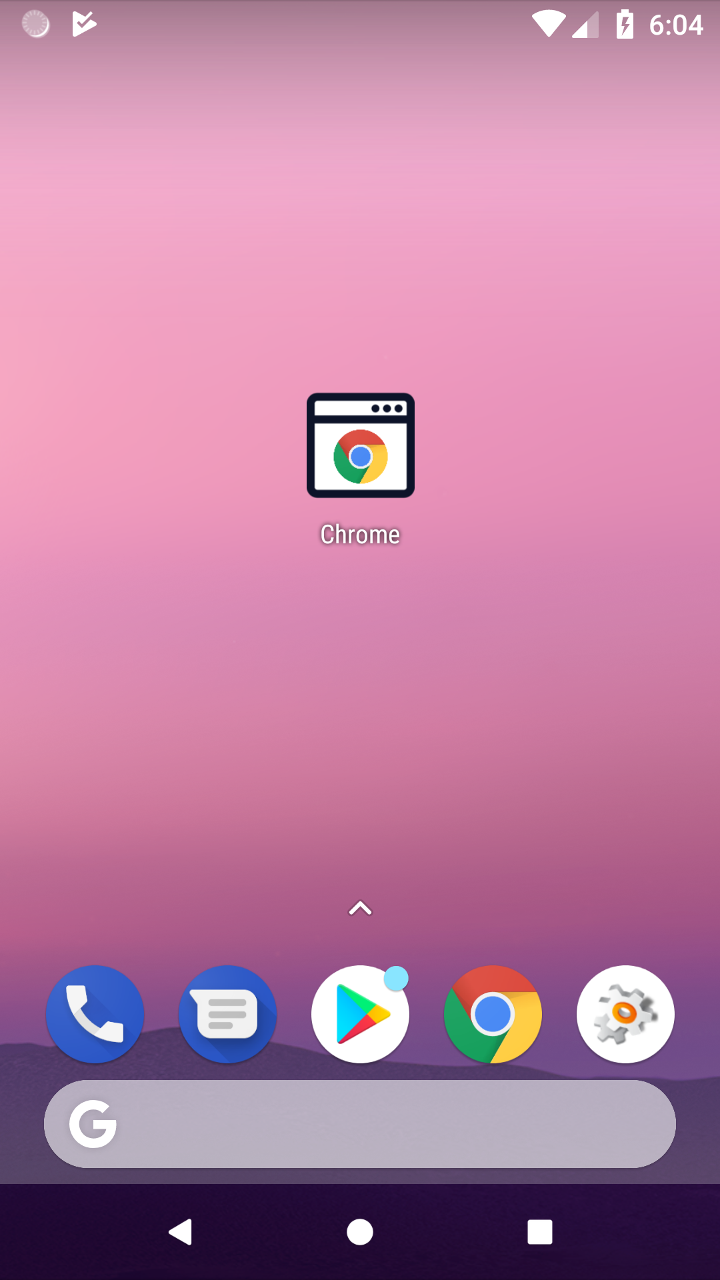This image showcases the home screen of an Android mobile device, specifically featuring a variety of app icons and system notifications. In the top left corner, the Google Play Store icon is prominently displayed, alongside a notification icon. The top right corner contains essential status indicators, including the Wi-Fi signal, network signal strength bars, battery charging indicator, and the current time, which reads 6:04. The home screen is populated with several app icons, including Chrome, the phone's dialer app, the Messages app, and again, the Google Play Store.